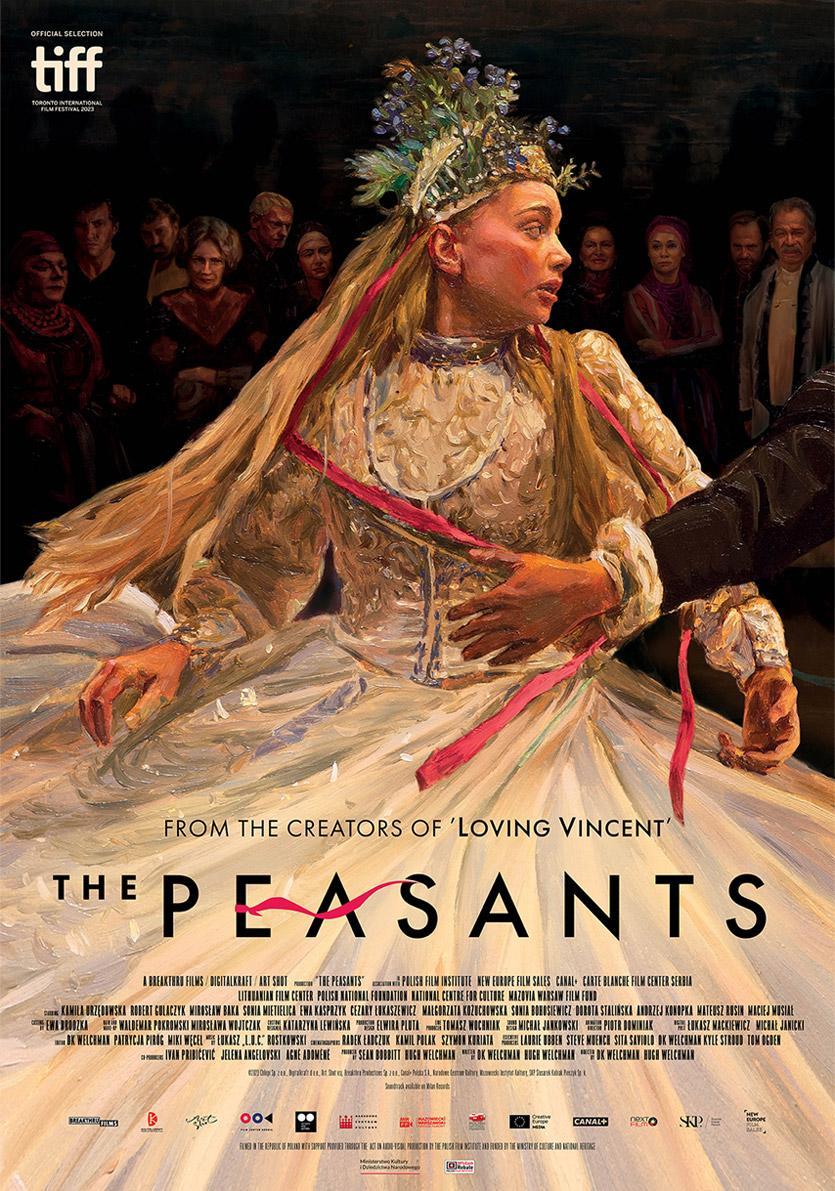This movie poster for "The Peasants," from the creators of "Loving Vincent," appears to have originated from the Toronto International Film Festival, as indicated by the TIFF logo in the upper left-hand corner. The artwork is rendered in a painterly style, not a photograph but with a highly detailed and artistic quality. The central figure, a distressed-looking young woman with blonde hair, is dressed in a glossy, white, full-skirted gown that features gold inserts and flows dramatically from her waist, taking up much of the bottom half of the image. She is adorned with a hat-like headpiece or tiara decorated with gaudy flowers and pink ribbons that cascade down. The scene captures her in mid-movement, possibly dancing or attempting to escape, as she appears to be looking over her shoulder, mouth open and looking distressed. A man's hand reaches from the side, grabbing at her waist as if trying to catch her in this dance or pull her back, echoing a sense of tension. In the background, a group of men and women with serious expressions look on, seemingly uninvolved in her immediate predicament. Across the title "The Peasants," a red scarf runs through the letters, visually connecting with the red ribbons in the woman's attire, tying the elements of the poster together.